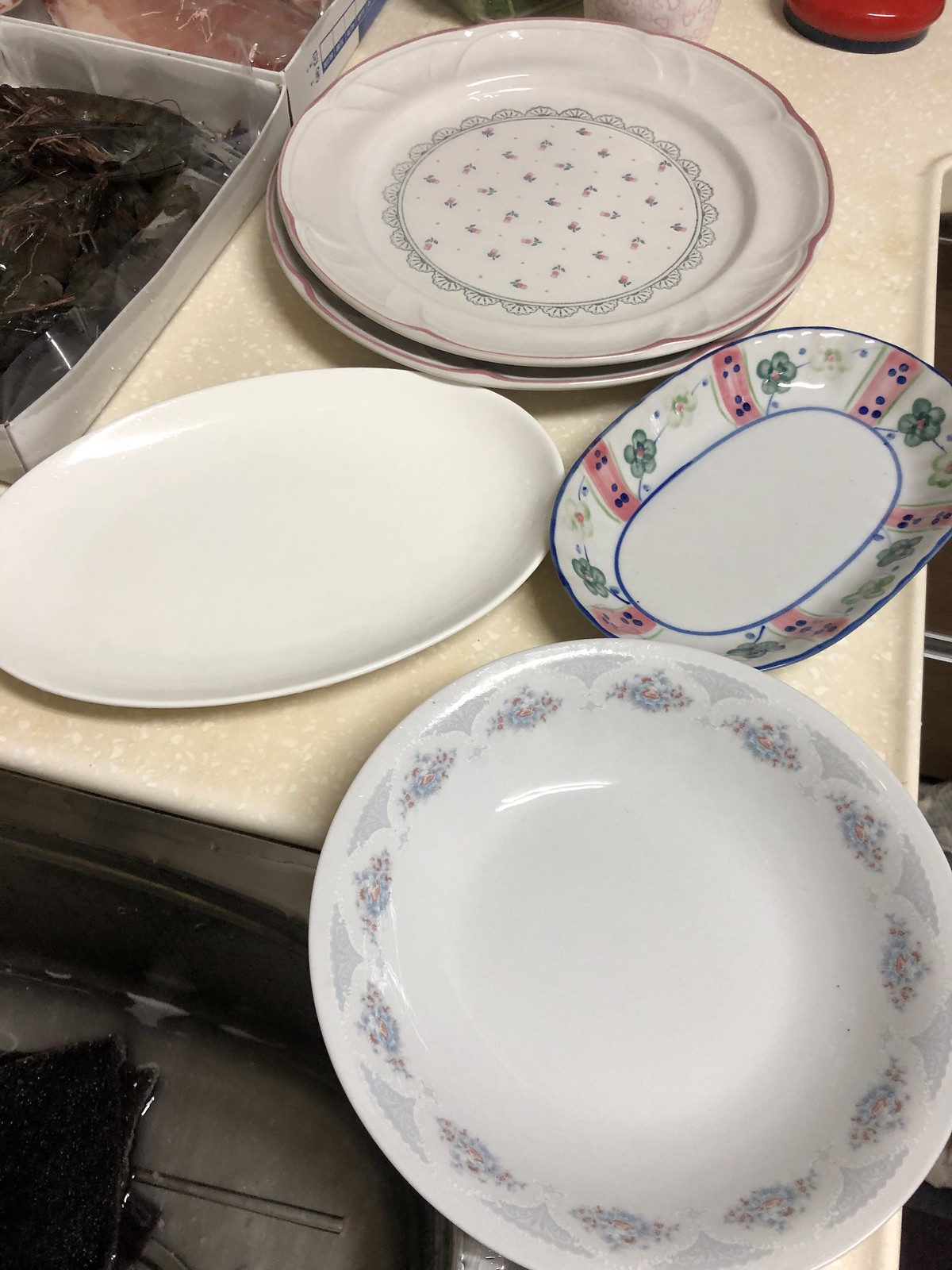The photograph captures a detailed arrangement of four distinct serving pieces on a cream-colored countertop that may have a slightly yellowish hue. Situated in the back are two circular dinner plates with intricately raised scalloped edges, accented by a thin pinkish-reddish line along the rim. These plates feature a gray central circle adorned with a grid of small flowers and a delicate lacy border around the inner design. Below these plates is a shallow, white circular dish with a geometric pattern of small flower bouquets around its lip. Positioned between the plates are two oval-shaped trays: one is plain white and seems suitable for small poultry, while the other boasts a decorative design with a blue oval at its base and along the outer edge, featuring painted flowers and vertical pink stripes interspersed with blue dots. In the upper left corner of the image, partially visible, are some silver or aluminum trays containing unidentifiable food items. The entire scene is set against a tan and white plastic surface, likely a kitchen countertop.